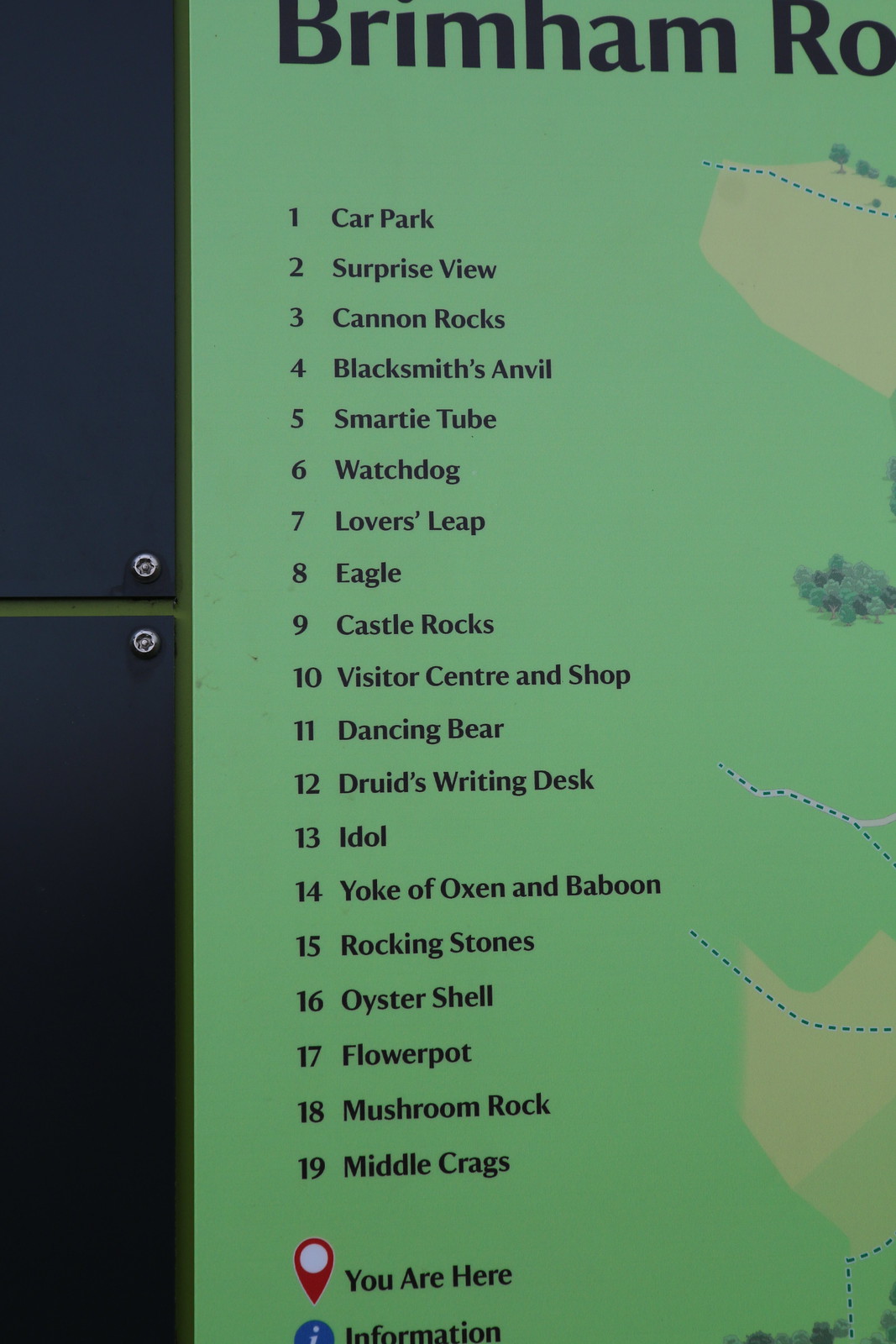This image focuses on the left half of a tourist information sign. The sign displays locations of specialty points of interest in a park, listed from 1 to 19. The background is primarily green, with text in black and navy blue. At the top, part of the sign reads “Brimham RO”, although the full text isn't visible. The list of destinations includes:

1. Car Park
2. Surprise View
3. Cannon Rocks
4. Blacksmith's Anvil
5. Smarty Tube
6. Watchdog
7. Lover's Leap
8. Eagle
9. Castle Rocks
10. Visitor Center and Shop
11. Dancing Bear
12. Druid's Writing Desk
13. Idol
14. Yoke of Oxen and Baboon
15. Rocking Stones
16. Oyster Shell
17. Flower Pot
18. Mushroom Rock
19. Middle Crags

Beneath this list, there is a red "You Are Here" indicator, with a blue "Information" marker below it. Part of the adjacent map is visible to the right, showing a green landscape with lighter yellow-green blotches and dotted trails, suggesting pathways. On the left side of the image, there are two large, square panels attached with screws, indicating this is an outdoor installation against a wall. The map features imagery of trees and a dotted line likely representing the trail network.